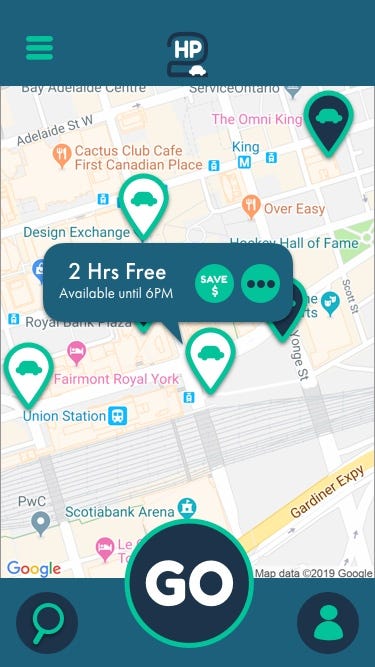A detailed description of the image is as follows:

The image displays a mobile application interface designed for car navigation or location services. The title of the application, "To HP," is prominently displayed at the top of the screen, overlaid on a dark green bar. To the upper left corner, there is a light green context menu icon consisting of three horizontal bars.

The central feature of the interface is a map that shows various notable locations in New York, New York including Union Station, Fairmont Royal Park, and Over Easy. These locations are marked clearly on the map. Text on the screen indicates that users can avail of two hours of free usage until 6 p.m., encouraging them to save cash through the provided context menu.

In the middle of the screen, there is a large green "Go" button, surrounded by a dark blue circle and outlined in white text, designed for initiating navigation or other primary actions within the app. 

At the bottom of the screen, there's a green bar featuring a search option on the left side, and a profile button on the right-hand side.

The design, color scheme, and placement of elements suggest a user-friendly interface aimed at providing navigation assistance and cost-saving options to its users.